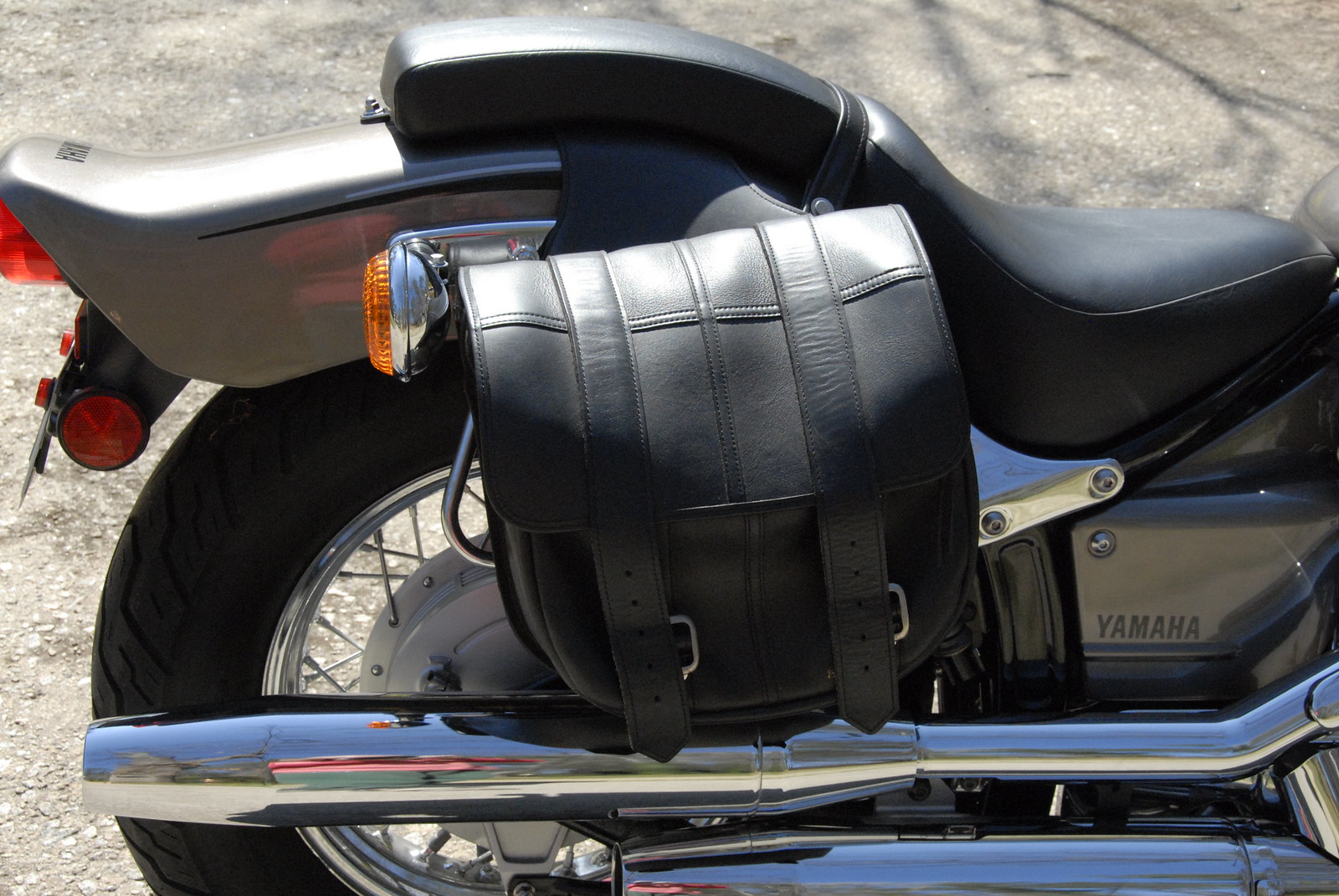This photograph captures the rear section of a Yamaha motorcycle. The image prominently features a large, black leather saddlebag with two belt buckles and straps that hang over the side, nearly touching the exhaust. The motorcycle, which appears to be a gray or champagne color, has a shiny, well-maintained look with an unworn black seat. The saddlebag looks new and is attached securely under the seat, which extends to the top right of the image. The "Yamaha" branding is clearly visible on the motorcycle's frame near the seat. The bike's back tire, silver spokes, and two reflective red lights are also in view. The scene is further accentuated by a large chrome exhaust pipe running along one side, likely glinting in the setting, which suggests it is situated in a dirt area with shadows indicating nearby trees.